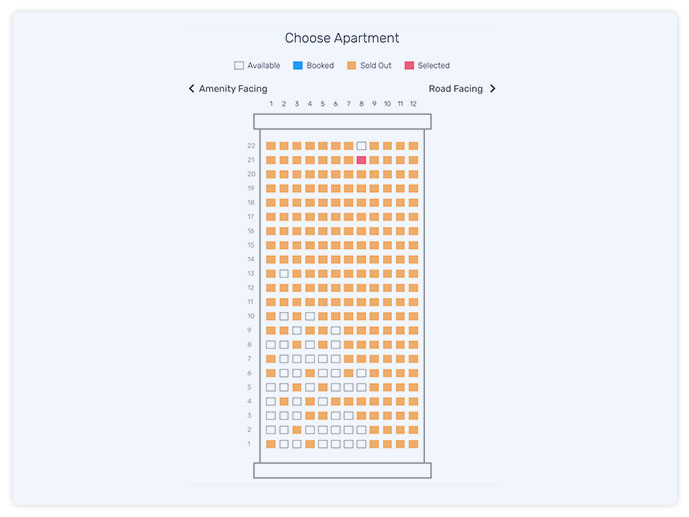The image is a detailed chart titled "Choose Apartment," designed to facilitate the selection of available apartments in a high-rise building. The chart includes a key for interpretation, where clear boxes represent available units, blue boxes indicate booked units, orange boxes show sold-out units, and red boxes highlight selected units. The columns are labeled from 1 to 12 across the top, while the rows indicate floors from 1st to 22nd, allowing for easy cross-referencing. The left side of the chart is labeled "Amenity Facing," and the right side is labeled "Road Facing," indicating the orientation of each apartment.

From the 14th floor upward, a significant majority of the units are booked, with the exception of a few key units. On the 21st floor, the unit in column 8 is available, positioned closer to the road-facing side but not quite halfway across. Additionally, an available unit can also be found on the 22nd floor, providing an option at the very top level of the building. This chart efficiently presents the current occupancy status of each apartment, aiding potential residents in making an informed decision.